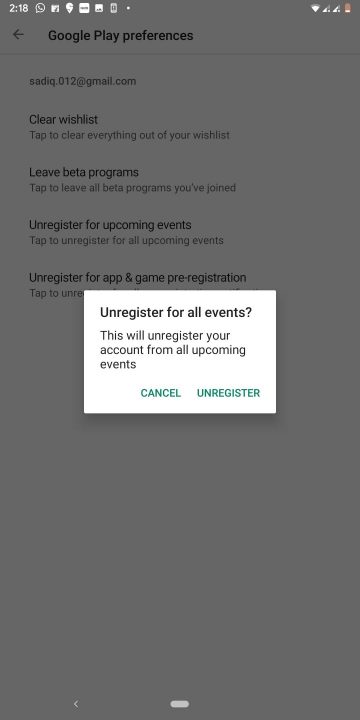A detailed screenshot of a phone screen is displayed. At the top, white text indicates the time as "2:18" along with a series of symbols including a WhatsApp icon. On the right side, additional icons appear, one of which is a vertical, red battery symbol. The majority of the screen has a dark gray shading.

Centrally, there's a prominent white box featuring bold black text stating "Unregister for all events?" Below it, regular black text explains, "This will unregister your account from all upcoming events." The box also contains two options in bold green uppercase text: "CANCEL" and "UNREGISTER."

Behind this white box, the gray background reveals additional information. At the very top, in bold black font, it reads "Google Play preferences," accompanied by a left-pointing arrow. Below it, the email address "Sadiq.012@gmail.com" is displayed. Further down, bold black text says "Clear wishlist," with an instruction in lighter gray text: "Tap to clear everything out of your wishlist." Continuing, bold black text reads "Leave beta programs," with a description in light gray indicating, "Tap to leave all beta programs you've joined." Finally, bold black text reiterates "Unregister for upcoming events."